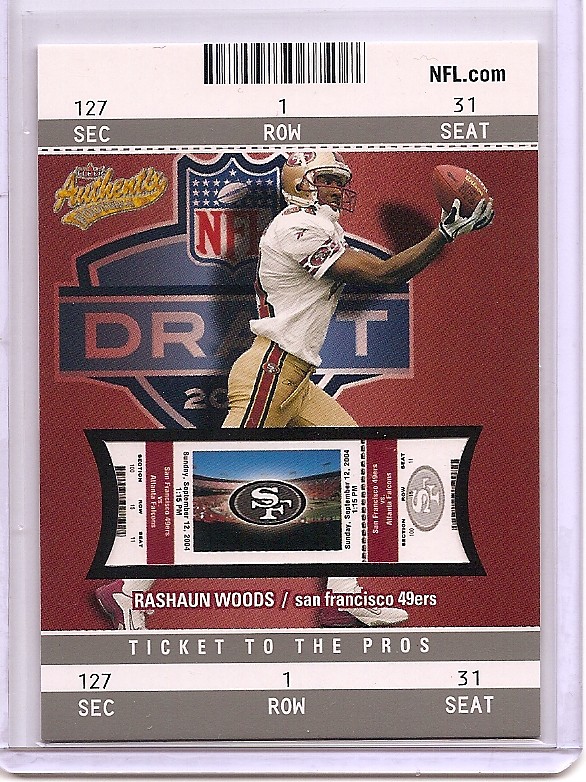This detailed image depicts a collectible football sports trading card encased in a plastic protective sleeve. The card features a simulated ticket design for a game, prominently displaying Section 127, Row 1, Seat 31 at both the top and bottom. At the top center, there is a barcode, with "NFL.com" in black lettering in the top right corner. The ticket details—"SEC 127, ROW 1, SEAT 31"—are clearly marked below. The background of the card is a dark red, featuring the "NFL Draft" logo with the NFL shield partially obscured by the player.

At the heart of the card is an action photograph of Rashawn Woods, a player for the San Francisco 49ers, captured mid-play while receiving a pass. Rashawn is dressed in a white jersey, gold helmet, and gold pants with red stripes, along with red and white footwear and white and black gloves. The bottom portion of the card includes text reading "Rashawn Woods / San Francisco 49ers" and "Ticket to the Pros." The card merges the aesthetics of a traditional trading card with the excitement and nostalgia of a game day ticket.